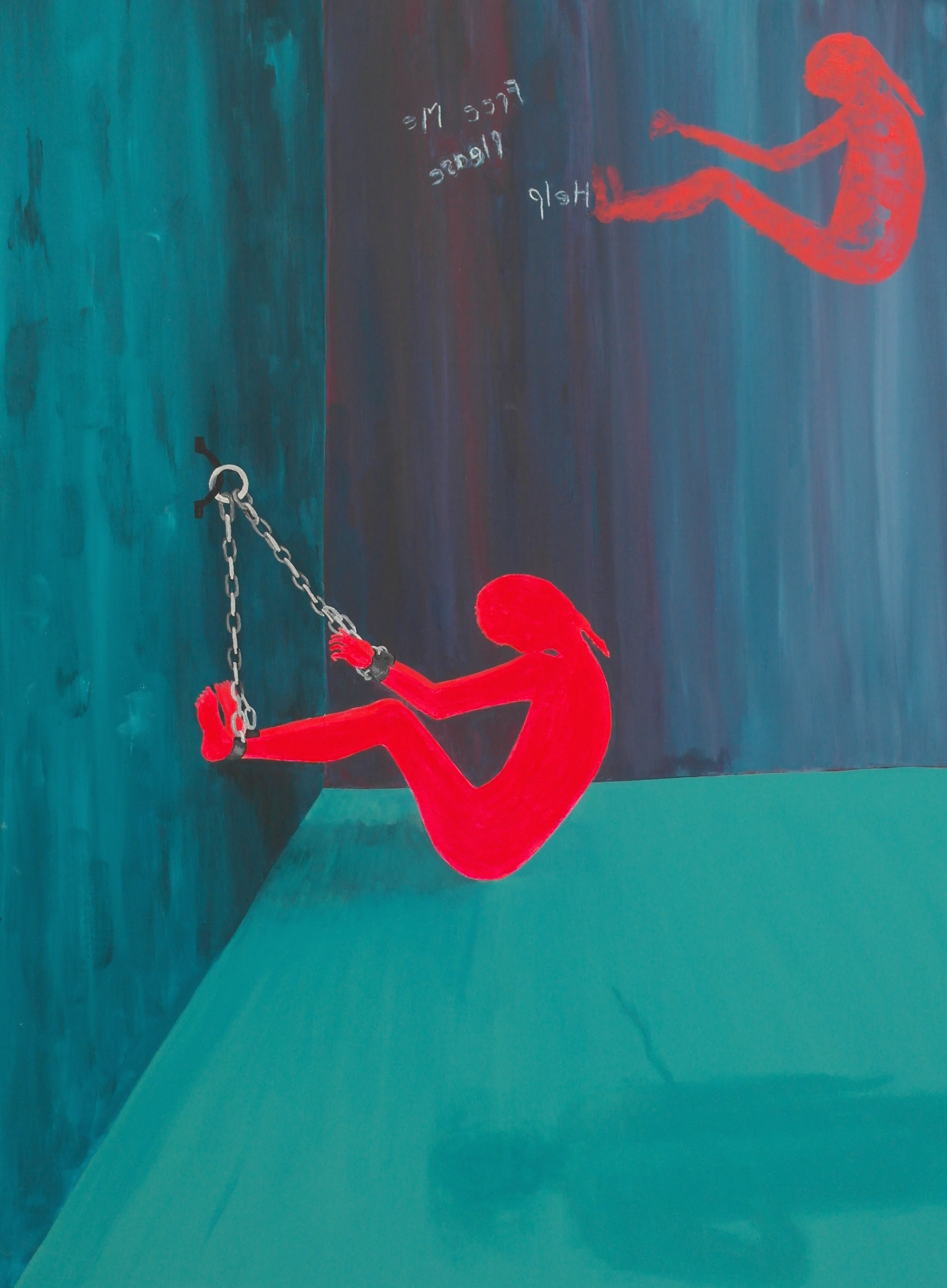The artwork is a haunting and twisted depiction of captivity, possibly in a cell within a prison or psychiatric ward. The scene features dark turquoise-blue, streaky walls with a dull blue floor. In the middle, there is a corner where the left wall is lighter in color than the right. 

Dominating the space is a red silhouette of a long-haired individual who is bound with silver chains, restricting their movement. The individual is seated with only their buttocks resting on the floor, while chains secure their ankles and wrists, lifting their feet about a foot off the ground and forcing their arm in front of them.

On the right-hand wall, almost suspended in a state of ethereal detachment, is another ghostly red silhouette drawn into the scene, possibly symbolizing the mental turmoil or haunting presence of the captive. 

Scattered scribblings and numbers like "97" and "999" are etched into the walls, contributing to the sense of desperation. Above, printed backwards in white letters, is a plea for help, reading, "FREE ME PLEASE HELP."

All elements in the piece stand upright, intensifying the confined and upright tension of the prison-like setting, making it a deeply emotional and unsettling visual experience.